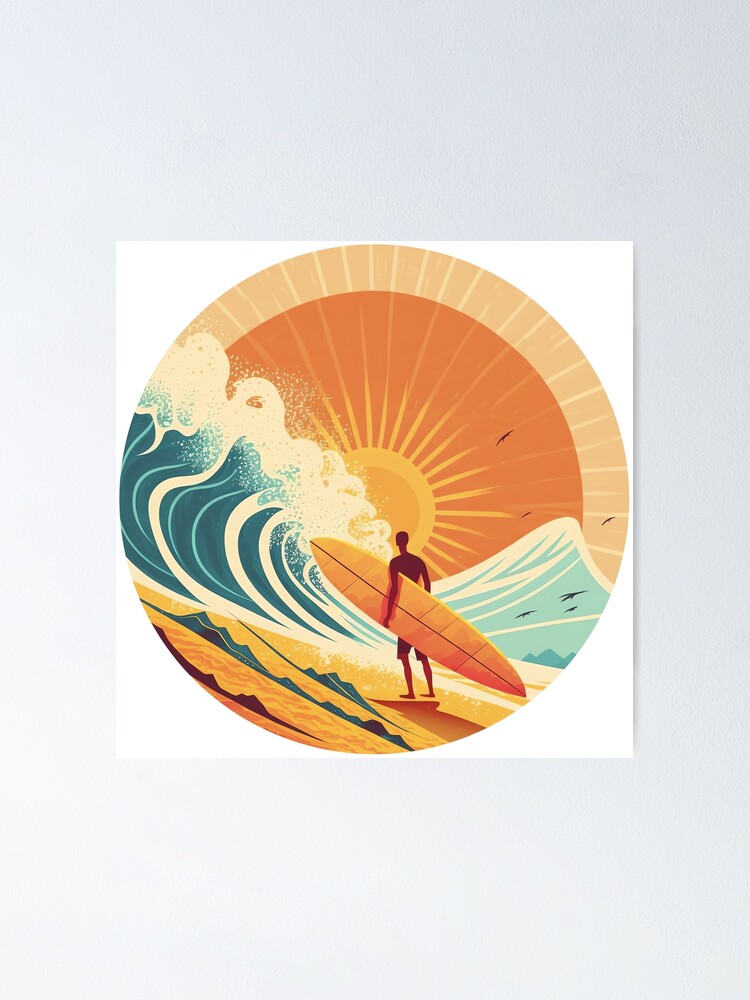The image is a detailed, art deco-style piece depicting a surfing scene, intricately framed within a square, white background. At the center of the circular artwork is a silhouette of a man in a brownish-red hue, holding a long yellow surfboard under his left arm. He stands on yellow-tan sand, observing a magnificent scene where stylized, blue and eggplant-colored waves rise prominently on the left and slightly on the right side of the circle. A large sun, partially obscured by white-capped waves, radiates muted coral-orange beams from the center, transitioning to an even lighter coral-orange near the top half of the circle. The waves create a dynamic contrast with their dark blue hues and triangular shapes, giving the impression of a powerful tidal wave receding into the ocean. The overall composition exudes a nostalgic yet vibrant energy, capturing a peaceful moment just as the sun is setting.